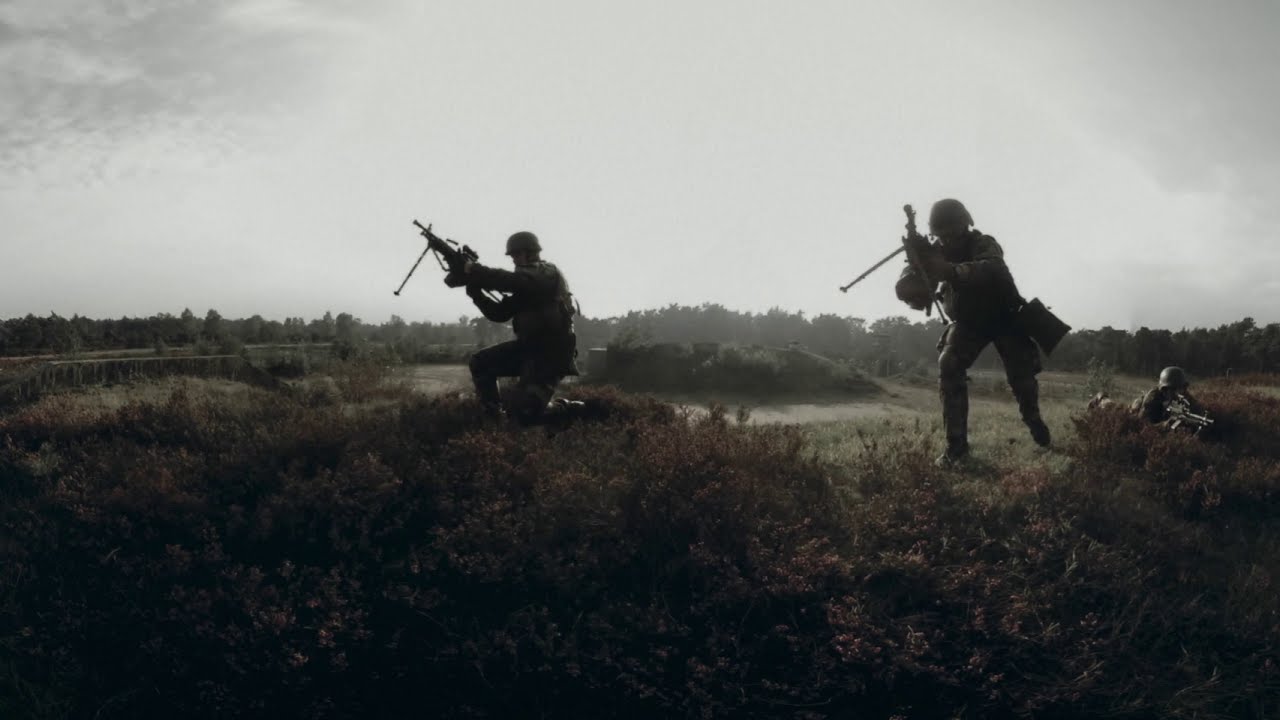The image captures a seemingly vintage scene reminiscent of World War II. At the center and right, a soldier is lying prone on the ground, aiming a machine gun amidst dense shrubbery. To his left stands another soldier, advancing with a large automatic rifle that features tripod legs for stabilization, a bag at his waist, and a helmet securely in place. Further to the left, another soldier kneels, also equipped with a similar type of rifle with tripod support, his weapon slightly raised. All three men are in full combat uniforms, complete with helmets. The rural, brushy terrain they are in includes a clearing surrounded by thick grass, bushes, and a tree line in the distance, with a body of water, perhaps a river or pond, visible behind them. The sky is partly cloudy with a hazy blue and white hue. The image, possibly in sepia or a muted color tone, has an artsy, shadowy quality, enhancing the dramatic and almost cinematic feel of the scene.